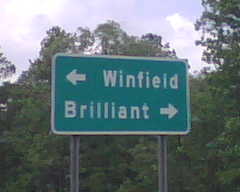In the image, there's a green directional road sign with white lettering and border, mounted on two gray poles. The top part of the sign features a white left-pointing arrow next to the name "Winfield" (or possibly "Winfeed"), with the letters clearly spelled out. Below this, another white arrow points to the right towards "Brilliant," with the exact spelling also provided. The background showcases a dense array of solid green trees, indicating a lush, verdant area. Above the sign, the sky is partially visible, exhibiting a mix of clouds with a slight purplish hue, suggesting an impending thunderstorm. To the bottom right of the sign, a noticeable black line extends, adding a distinct visual element to the scene.